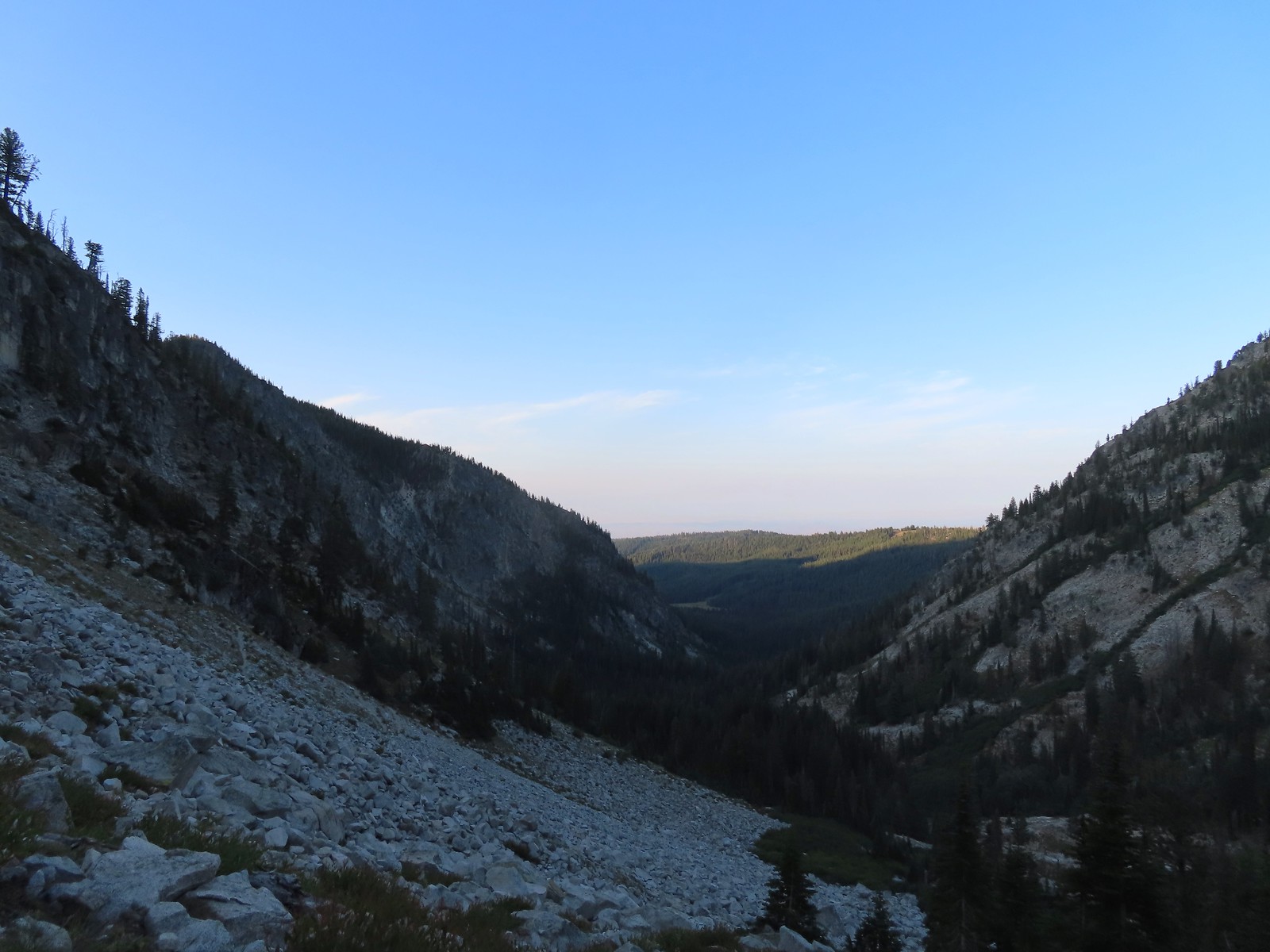In the picture, a stunning valley stretches out between two large, rocky hillsides that converge into a picturesque vista. The valley floor is shaded, with limited sunlight adding a slightly darker tone. Both hillsides are speckled with chunks of white rock and gravel, some appearing pulverized into smaller pieces. Among the rocks, several pine trees manage to anchor themselves in the crevices, painting a rugged yet lush landscape. The valley floor is densely blanketed with evergreen trees, possibly accompanied by a flowing stream and small green patches of fields that break the monotony of the tree cover.

In the background, the valley opens up to reveal another mountain range, which is abundantly green and covered with a thick, verdant blanket of trees. The sky above is a clear, deep blue, hinting at a pending sunset that casts shadows over the hills. The subtle play of light and shadow adds a rich texture, clearly depicting the valley's depth and the majestic, contrasting heights of the mountain ranges. The scene projects a serene yet dramatic natural beauty, drawing the eye from the rocky, tree-lined hillsides to the distant, green hills gently caressed by the fading sunlight.